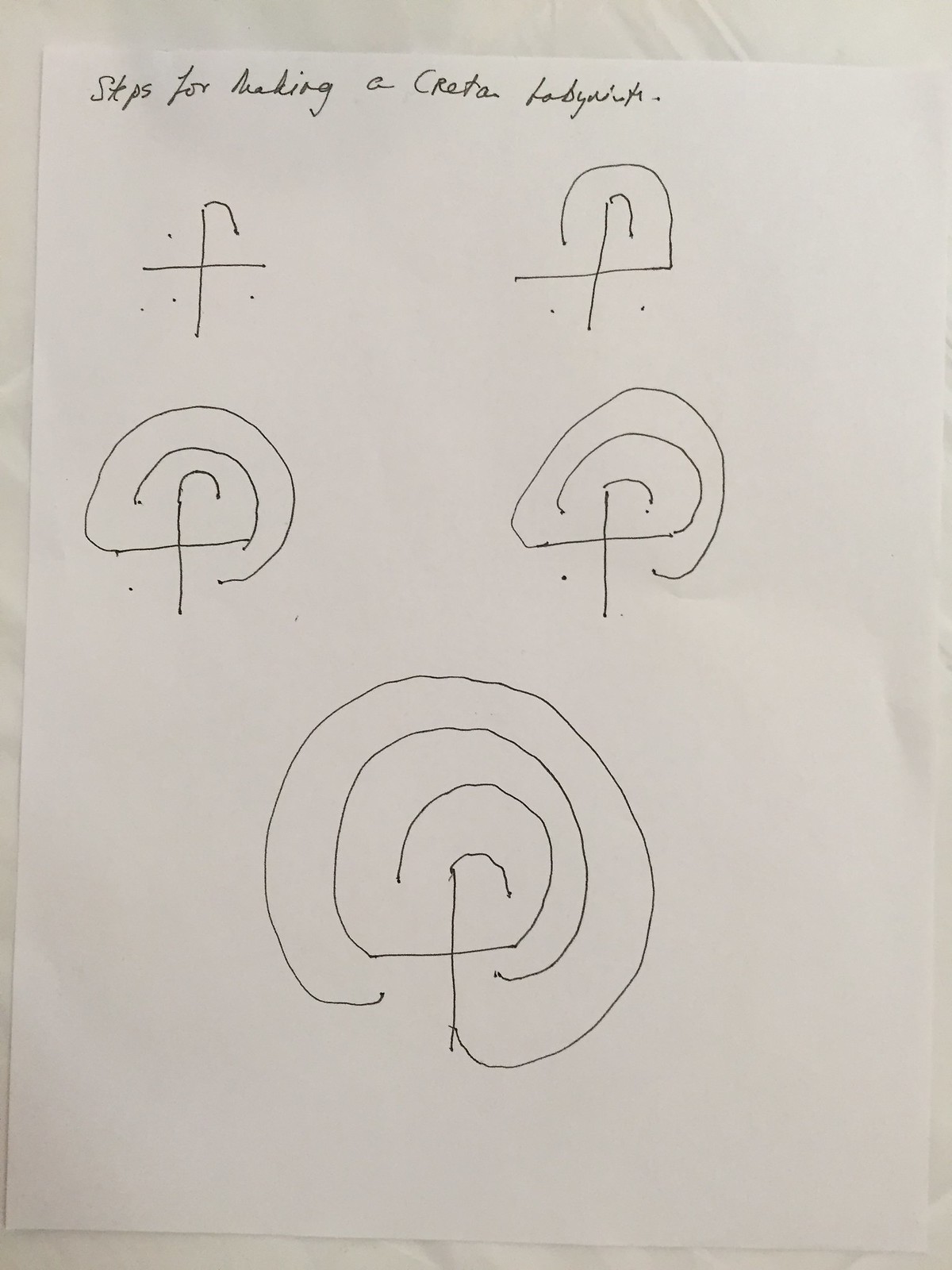The image captures a white sheet of paper placed on what appears to be a white table. The paper features a series of intricate drawings, all created using a black pen. At the top of the paper, cursive text reads, "Steps for making a creda," though the exact wording is somewhat difficult to decipher, possibly spelling out "L-O-B-Y-R-I-T-H."

The drawings begin with a circle encompassing them. On the top left, there is a plus sign with dots at each intersection. From the top of this plus sign, a curved line starts to form a partial circle. To the right, another drawing shows a semicircle extending from the far right end of a central horizontal line, curving up to the midpoint on the top left side.

Progressing to the third drawing, we see a dot originating from the far left end of a vertical line, which curves around to touch the bottom right midsection. The subsequent drawings showcase similar partial circular decorations around central lines and dots. 

In the final drawing, all circles are completed without any intersecting lines or dots, presenting a clean and comprehensive diagram of complex circular patterns.